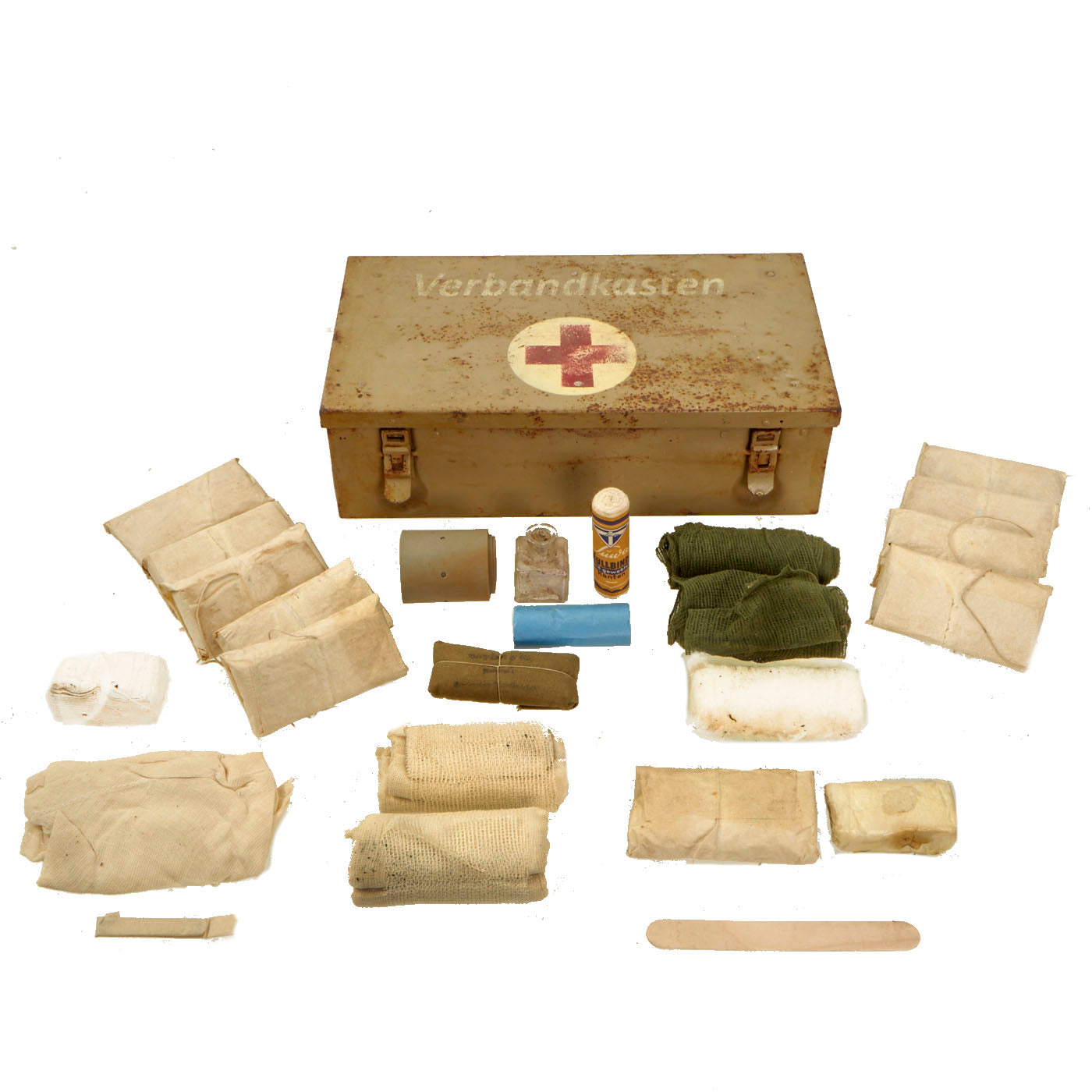The photograph captures an old-fashioned German first aid kit labeled "Verbandkasten" in white lettering. The weathered, metal box, adorned with a circular emblem featuring the universal Red Cross symbol, hints at extensive use. The kit's rustic and dented exterior is secured with metal clasps. Displayed meticulously in front of the box, as though in a museum exhibit, are its various medical supplies. Among these are gauze, bandages, cloth pieces—some green—and what appears to be a popsicle stick for medical examinations. Included are items such as tape, a bottle of iodine, an orange-labeled powder container, and band-aids, all laid out on a white background to highlight their historical significance.